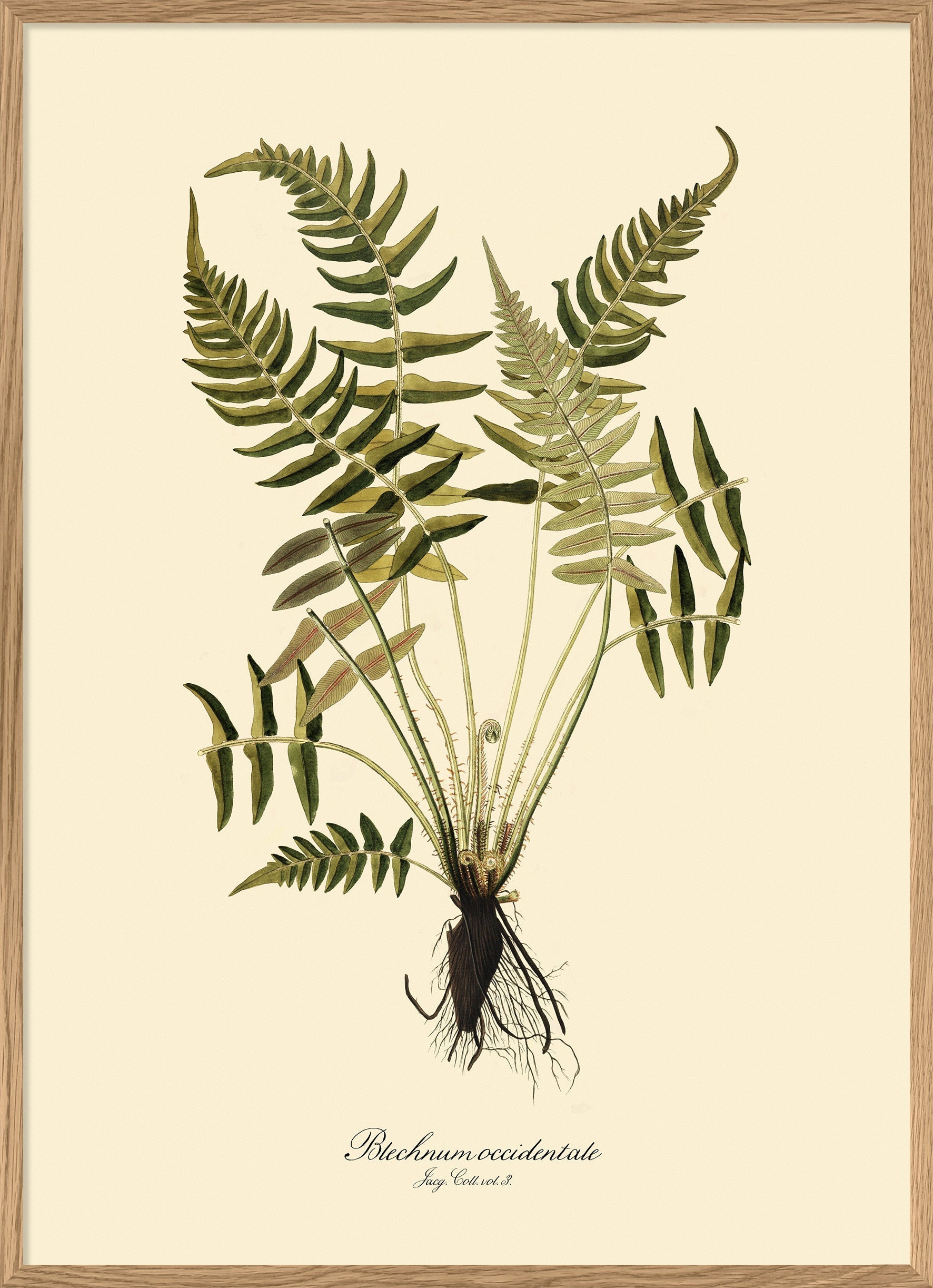The image depicts a framed painting of a unique plant species, "Birch Monocan," set against a pink background. The frame is made of wood with a brown color, giving it a rustic appearance. The central background of the image is green, enhancing the plant's intricate details. The plant itself resembles the form of a dancing insect or a woman's body, characterized by its curves, round eyes, and raised "arms." Its roots extend like black branches, with green leaves sprouting from the stems. At the bottom of the painting, there is a label that reads "Birch Monocan," marking it as the species name. The overall effect is both artistic and detailed, highlighting the plant's stems, roots, and leaves with significant height.